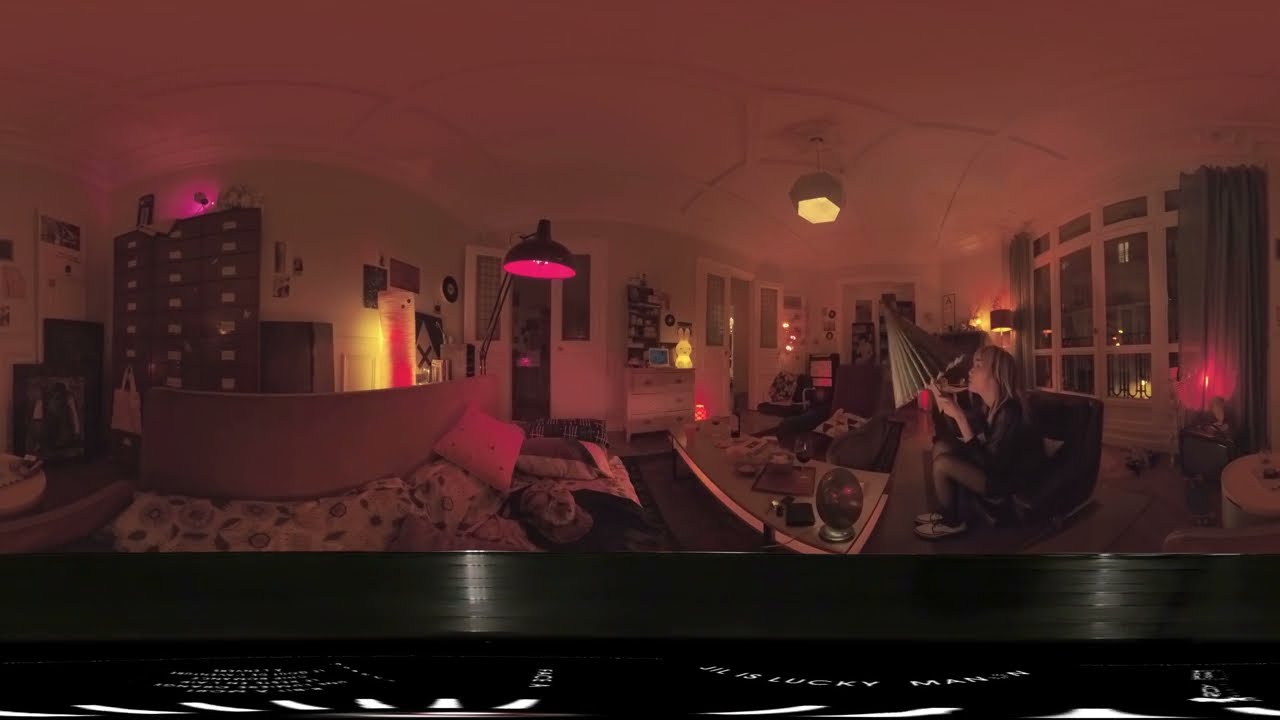In this dimly lit, panoramic nighttime photograph of an apartment, the scene centers around a woman with blonde hair, dressed in black, sitting on a black leather armchair in front of a four-pane window with white frames and green curtains. She holds a heavily opened green umbrella. The room, painted in white with matching ceilings, contains various furniture and decorations. In front of the woman is a white desk cluttered with several items, beyond which lies a bed or couch, covered with a white patterned blanket and topped with two pillows, suggesting a possible studio apartment setup. The ambient lighting includes a pink ceiling lamp, a yellow lamp hanging near the window, and a reddish floor lamp that collectively cast a warm, reddish undertone throughout the space. Cabinets or shelves filled with knickknacks and objects line the left side of the room, contributing to the eclectic and unique atmosphere. Through the window, a cityscape hints at urban living.